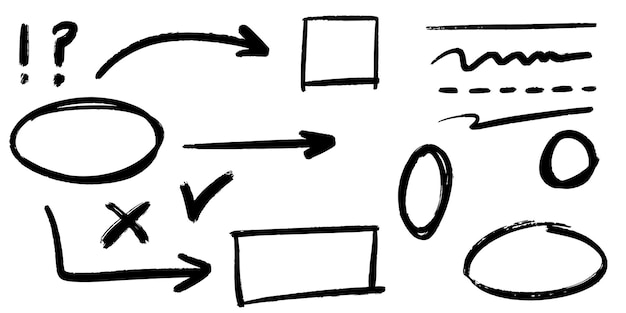The drawing is a complex series of black marker illustrations on paper. On the right-hand side, there's a horizontal line, a squiggle, a dashed line, and what looks like an almost checkmark shape that also resembles a child's drawing of a seagull. There are also three large shapes: two ovals and one circle. 

In the center, slightly to the left of these shapes, a square is positioned at the top with an arrow pointing to the right. Below this, there is a rectangle. 

On the left third of the drawing, in the top right-hand corner, there is an exclamation point and a question mark. There is also an oval with a swooping mark connecting it to the square. An arrow in an L shape points downward and then towards the rectangle, giving the impression of a flowchart. Between the oval and the rectangle, there are an "X" and a checkmark.